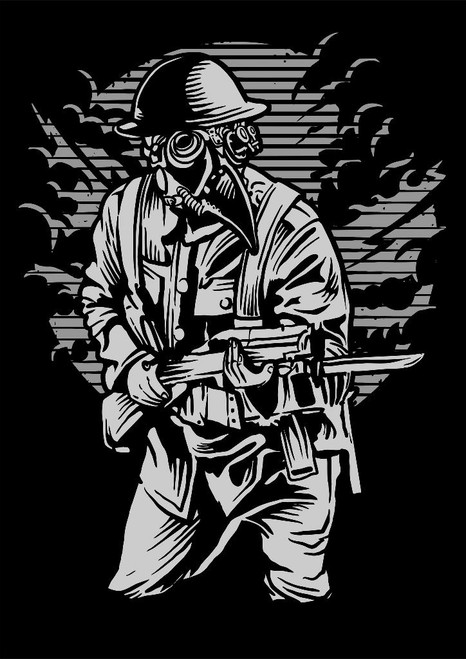The black and white drawing depicts a dystopian-looking soldier set against a black background. At the center of the image, the soldier stands with his lower half ending at the knees, his feet not visible. Encased in a bird-like gas mask, which features a beak and large, menacing eyes, he looks to the right. A brimmed hat tops his head. His attire includes a long-sleeve, button-down jacket with chest pockets and front pockets, baggy pants, and suspenders crossing over his shoulders. He clutches a rifle close to his body, which is fitted with a bayonet. Detailed with a belt buckle, his uniform adds to the menacing presence. In the background, a light gray, rough-edged circle, possibly suggesting a torn paper or smoke, contrasts with the dark vertical stripes within. The entire scene gives a stark and eerie ambiance, enhancing the soldier's grim and foreboding appearance.